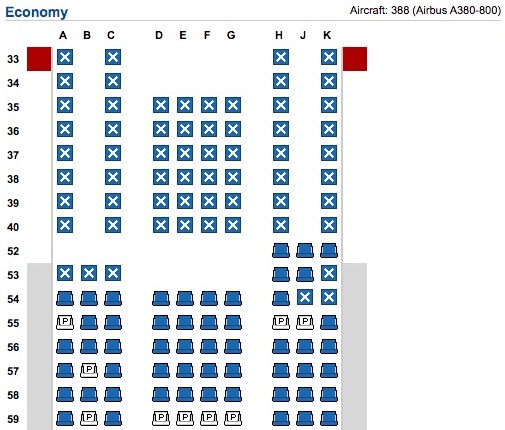This detailed seating plan is for an Airbus A380-800 aircraft. The seats are organized in rows labeled with numbers ranging from 33 to 59 on the left-hand side, while columns are marked with letters A, B, C, D, E, F, G, H, J, and K. This configuration allows the plane to seat a substantial number of passengers.

The seating map displays three types of seats: blue seats, which are available for selection; seats marked with the letter 'P'; and seats crossed out with white X's, indicating they are already taken. Additionally, there are two small red bars located in the upper left and right corners of the map, though their purpose is not specified.

This map appears to depict the economy section of the aircraft, as indicated by blue lettering in the upper left corner. The majority of the plane's rear section is shown, with the central rows comprising 20 seats each, while the two side sections consist of 14 seats each. Most seats in this section are already occupied, demonstrating the high capacity and popularity of this Airbus A380-800's economy class.